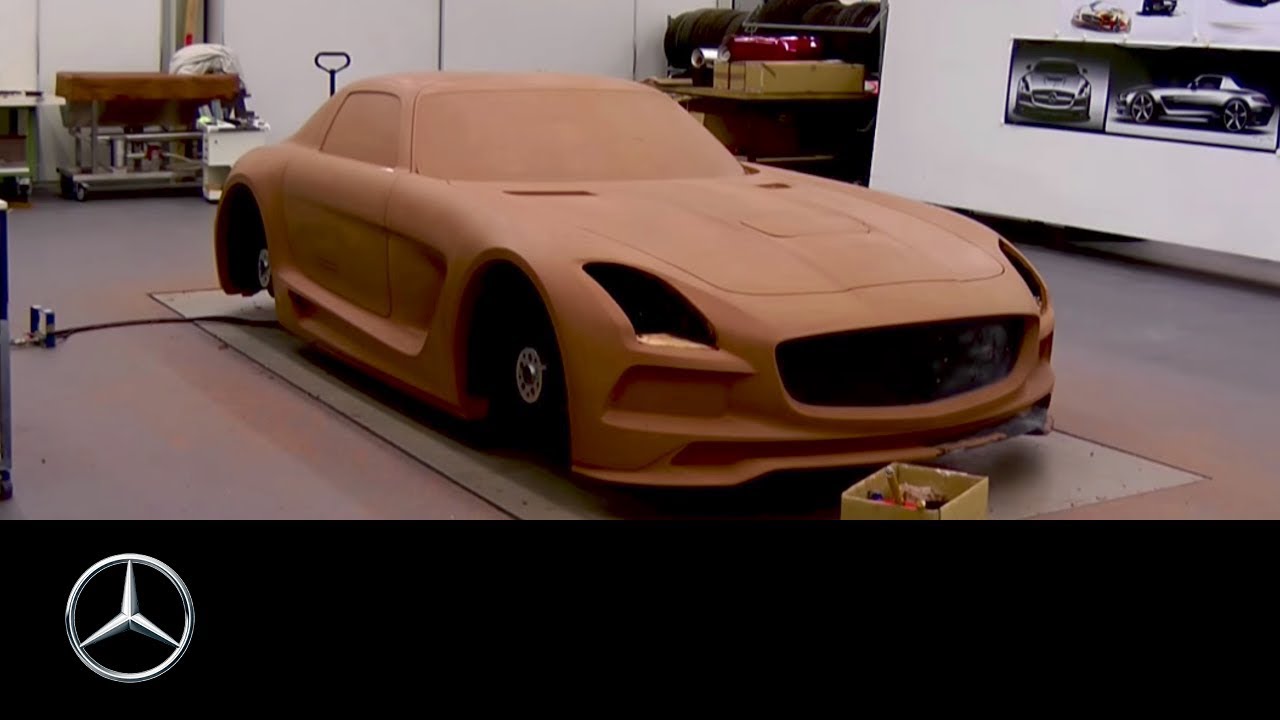This detailed photograph captures an automobile prototype located in what appears to be an automotive workshop. The prototype, a sleek luxury sports car, possibly a Mercedes, is sculpted in a clay terracotta or light brown color that completely envelops it, including the windows. Notably, the car lacks essential details such as headlights, wheels, and a front grille, indicating it is in the early stages of development. 

The setting is a sparse workshop with a floor that seems to be either a copper-iron or lighter purple, dark gray hue. The room features a pushcart with some indistinct tools, a yellow box in front of the car, and a workbench in the background. On the upper right, a white wall displays photographs or 3D renderings of what the finished automobile might look like, showcasing a polished chrome or black version of the car.

At the bottom of the image, a distinctive black bar runs across, empty except for the far left corner, which features a three-pointed star logo within a steel circle, suggesting Mercedes branding. However, one of the descriptions also mentions a Mitsubishi logo, potentially indicating some confusion or error in the setup. Posters of various cars further decorate the wall, reinforcing the automotive theme of the workspace. The car's sleek and unfinished form, combined with the industrial backdrop, vividly depicts the meticulous process of car design and prototyping.